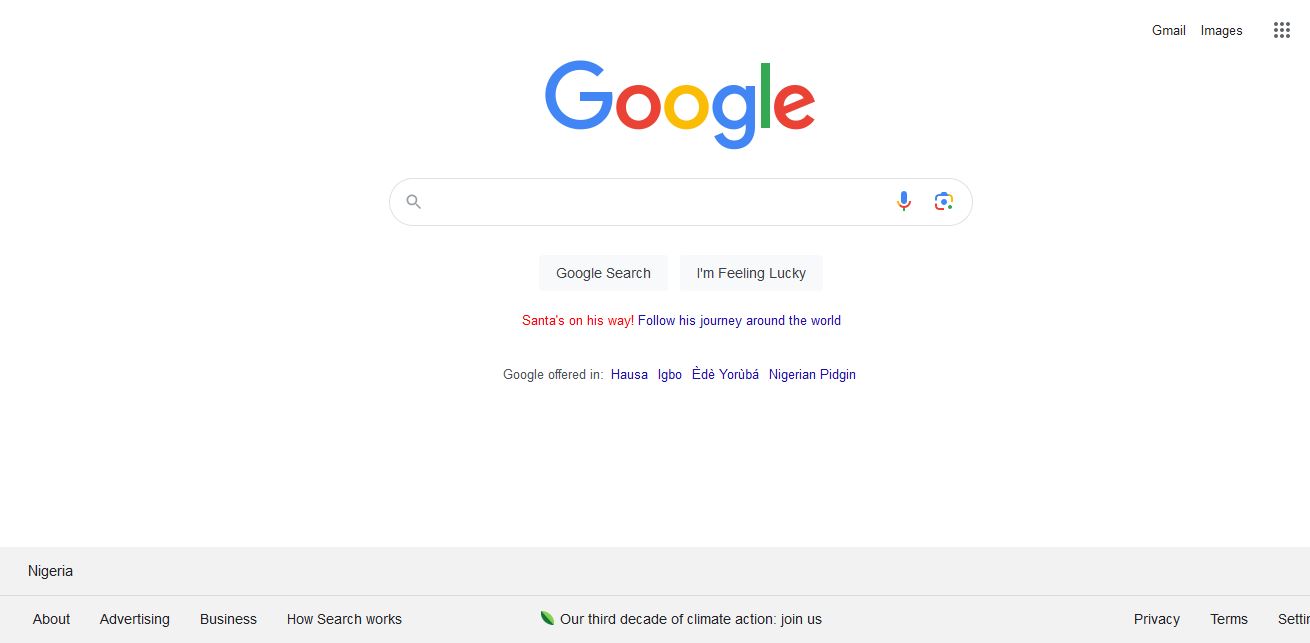This is a left-to-right horizontal image captured from a digital device, likely a smartphone or computer. The image appears to be a screenshot of an open webpage. The background is predominantly white, presumably the color of the webpage itself.

In the upper right-hand corner, the words "Gmail" and "Images" are displayed in black. Next to these, there is a small icon featuring a grid of dots, which is a common representation for accessing additional Google apps.

Dominating the center of the page is the iconic Google logo, with a search box positioned below it. The search box contains the familiar magnifying glass icon, a microphone icon, and a photo icon. Beneath the search box, there are two clickable buttons labeled "Google Search" and "I'm Feeling Lucky."

In vivid red text beneath these buttons, a festive message reads, "Santa's on his way." Below this, in blue text, it says, "Follow his journey around the world." Further down, the text mentioned that Google is available in different languages.

At the very bottom of the page, there is a long, gray rectangular bar that shares various links such as "Nigeria," "About," "Advertising," "Business," "How Search Works," "Our Third Decade of Climate Action," and "Join Us." To the right of this bar, additional links for "Privacy," "Terms," and "Settings" are displayed.